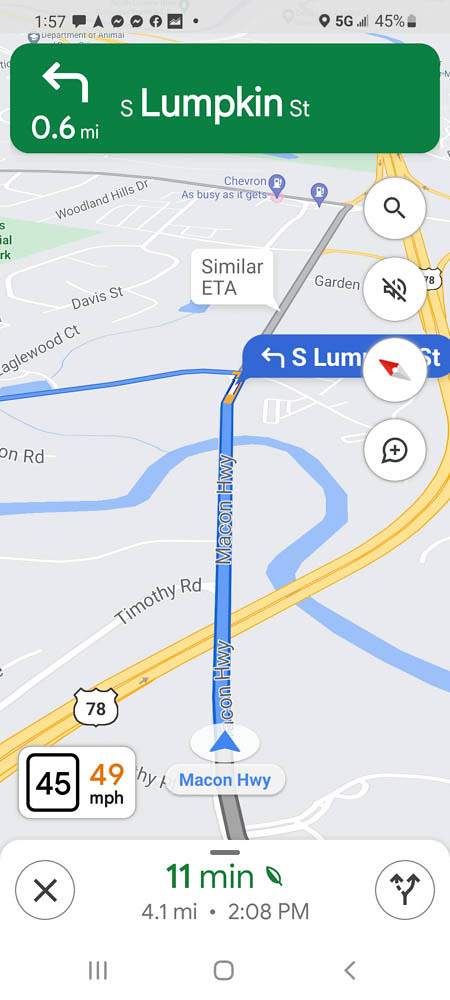A detailed screenshot from a Google Maps navigation session on a smartphone, showing a user traveling on Macon Highway at 49 mph in a 45 mph zone. The navigation interface at the top indicates the next turn in 0.6 miles, a left turn onto South Lumpkin Street. At the bottom, the display reveals 11 minutes and 4.1 miles remaining to the destination, with an estimated arrival time of 2:08 p.m. The current time, displayed at the top left, is 1:57 p.m.